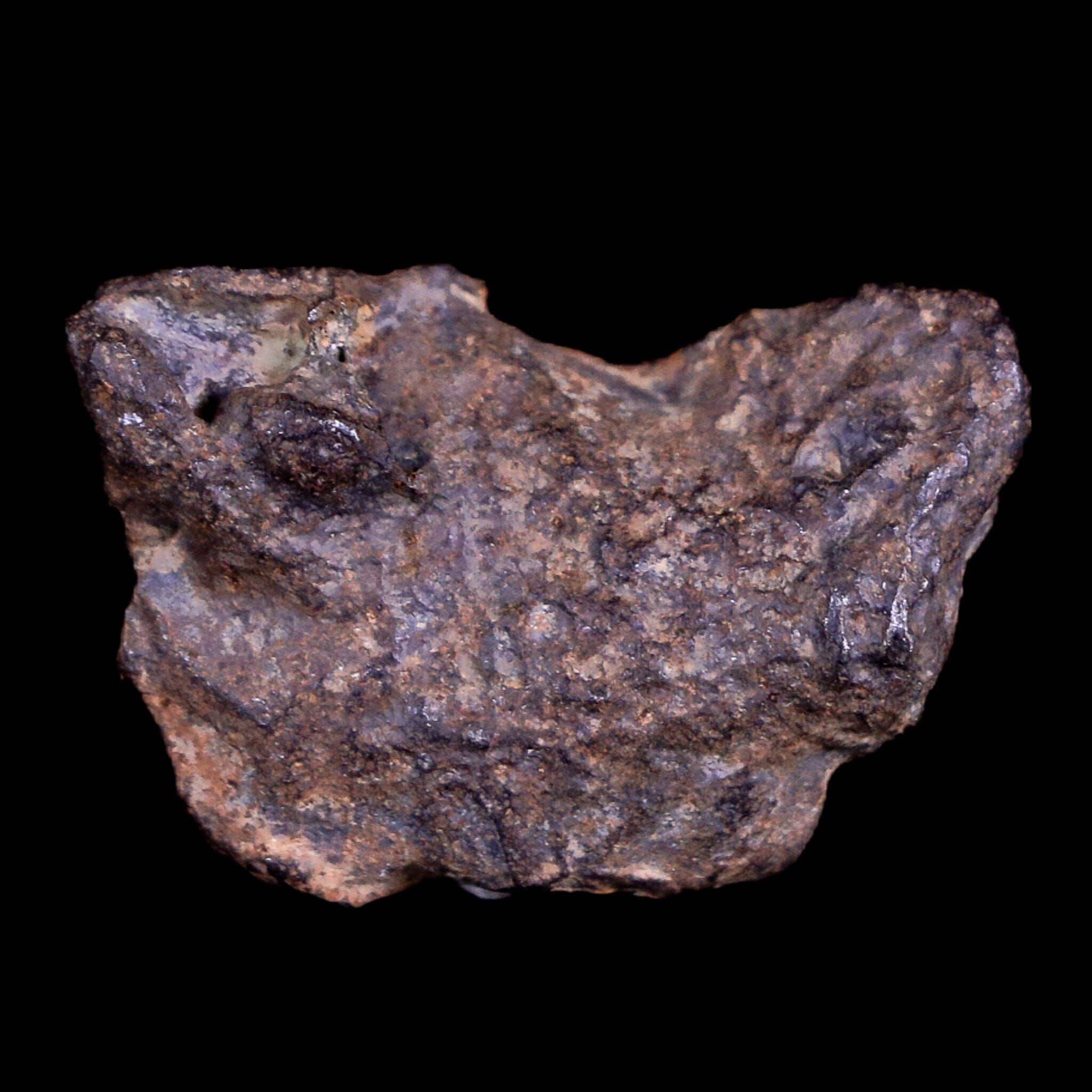The image features an irregularly shaped rock or meteorite-like object, predominantly brown in color with varying shades of brown and interspersed with black spots. It has a unique form reminiscent of a squat frog's head or a 'W' without the legs, with distinct protrusions on the top left and top right sides, and a notable dent in the middle. There are two prominent holes or oval-like indentations on the top left and top right that resemble eyes, contributing to the rock's distinctive appearance. The base of the rock is narrower compared to its top, and its surface shows some shiny aspects, especially on the right side. The object appears to be floating in space against a completely black background.